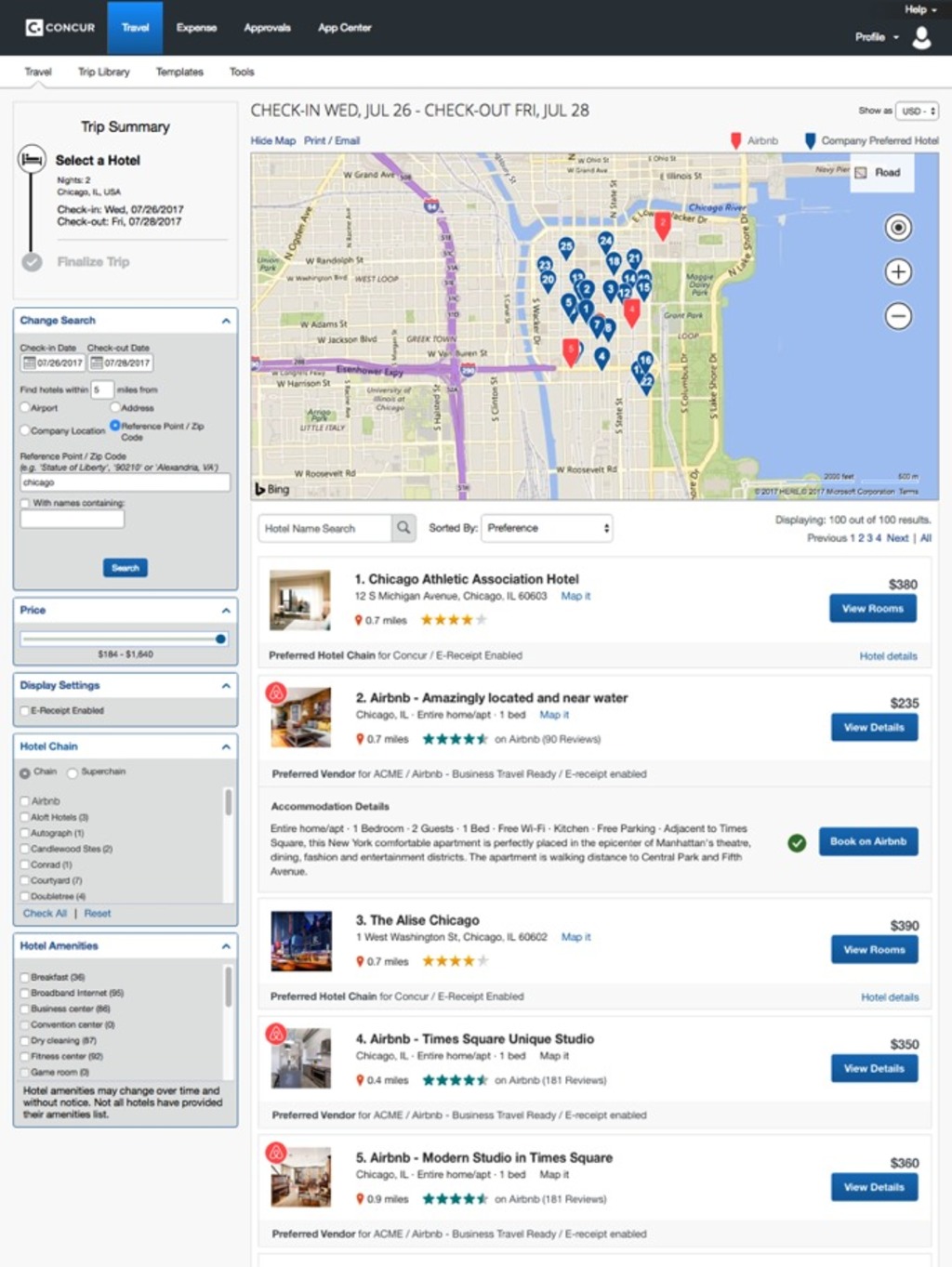This is a detailed screenshot of a travel website's interface. The top of the webpage features a prominent blue banner with the company's logo located on the upper left corner. Adjacent to the logo are four navigational sections, among which the "Travel" section is highlighted in light blue for better visibility. 

On the left side of the page, there is a narrow vertical panel. At the top of this panel, there is a box labeled "Trip Summary." Directly beneath it, the text instructs users to "Select a hotel as the first step," followed by a dropdown search box for hotel selection. Below this are two additional dropdown boxes designed for inputting travel dates. Along the bottom of this panel are various categories, though part of it appears to be cropped due to the limited length compared to the main web content on the right.

Dominating the right side of the webpage is a large interactive map with numerous blue and red pin drops, indicating different locations. Beneath the map, there is a vertical list of hotels. Each hotel listing includes a thumbnail image on the left, the hotel's name and details in the center, and the price on the far right. Below the price, a blue bar labeled "View Rooms" invites users to see more details about the available accommodations.